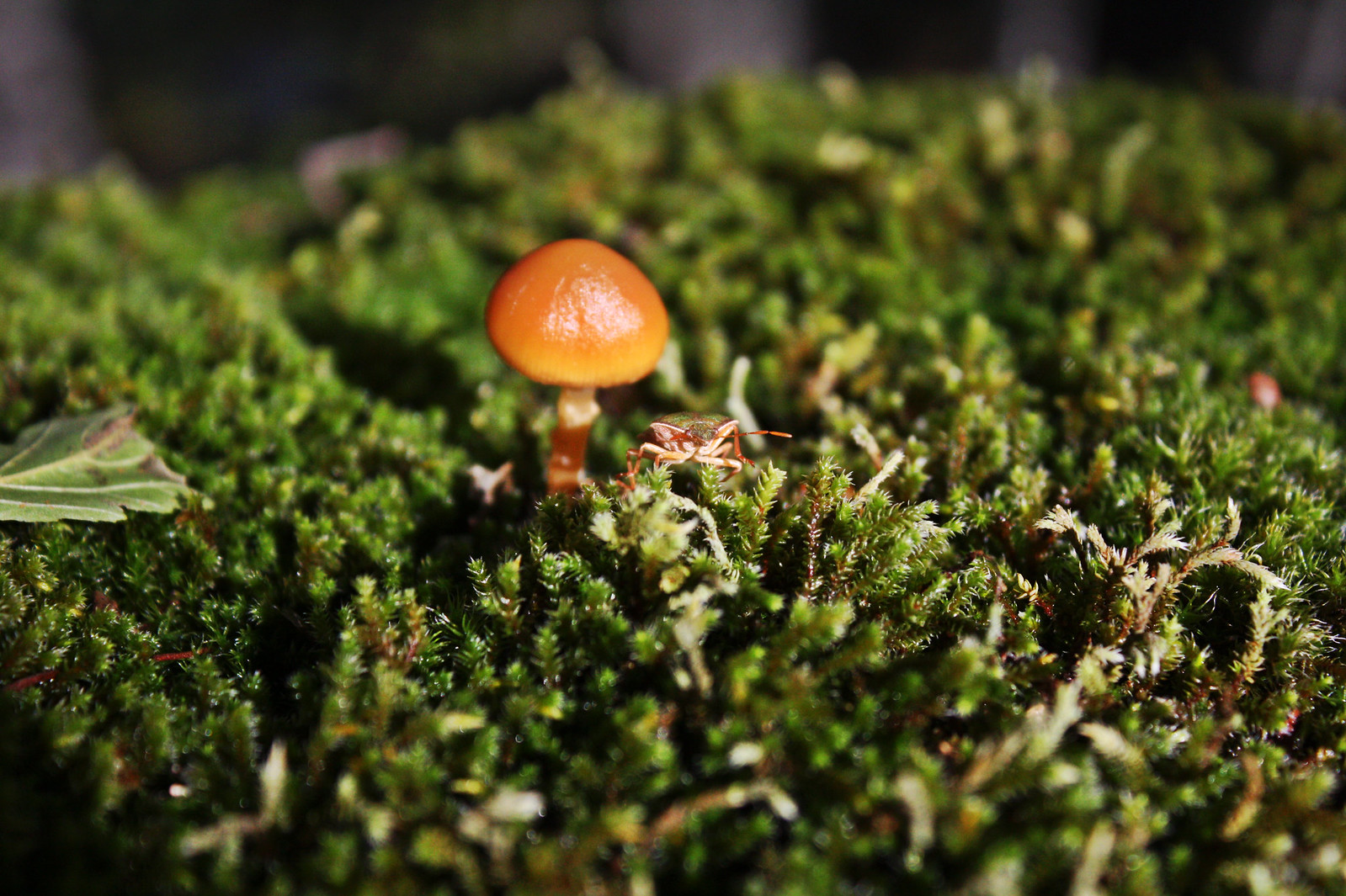The image depicts an extreme close-up of a tiny, bright orange mushroom with a small stem sprouting from the ground covered in lush green plants, resembling moss more than grass. The mushroom's vibrant orange cap contrasts sharply with the greenery around it. To the mid-left of the photo, a small green leaf is visible. The background is blurry, appearing in shades of black, brown, and gray, with subtle hints of yellow and blue. Illuminated by a light source, both the mushroom and the surrounding green plants are highlighted clearly. Adjacent to the mushroom, an insect, possibly a cockroach, is present. The insect's body blends with the green surroundings, its brown legs and antennae extending visibly. The overall scene captures the intricate details of the small mushroom and its immediate environment, emphasizing the vivid colors and close-up nature of the shot.